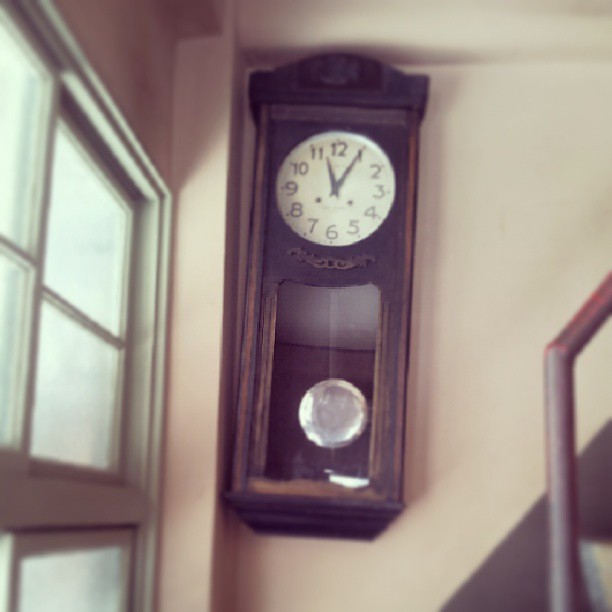This color photograph captures a beautifully detailed scene focused on a large, traditional pendulum wall clock, prominently displayed at the corner of a wall. The clock is encased in an intricately crafted, dark hardwood cabinet, suggesting that it might be an antique piece. The intersecting wall features part of a window, adding a touch of natural light to the setting. The clock boasts a classic white face with regular Arabic numerals, rather than Roman numerals. The hour and minute hands are sleek and black, and the time displayed is precisely 11:05. The clock’s pendulum, strikingly silver and polished to a bright shine, catches the ambient light, adding a gleaming focal point in the image.